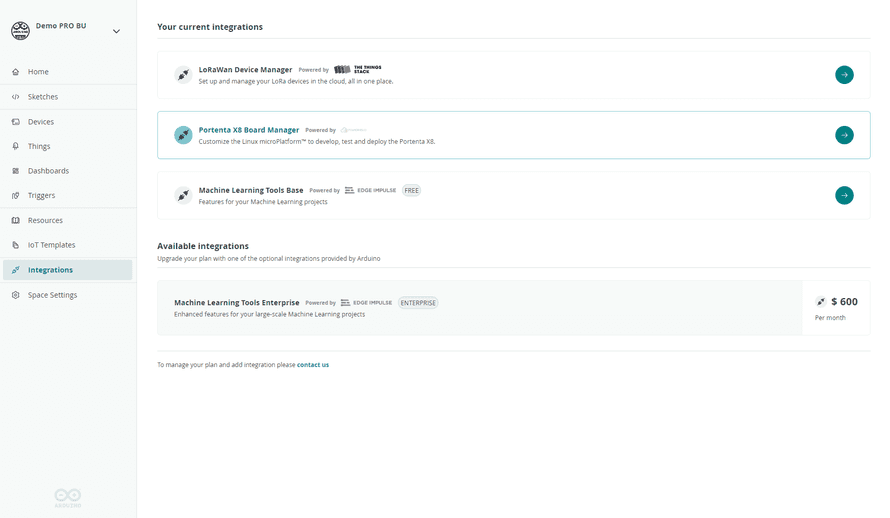**Caption: Detailed Overview of DemoProBU Interface**

The image showcases the interface of a computer program or website named DemoProBU. The main content area displays a section titled "Current Integrations," highlighting various available tools. Featured prominently are "Loran Device Manager," "Parenta XS Board Manager," and "Machine Learning Tool Space," with the latter marked as a free option. The other tools are described as "Powered by" specific companies. 

At the bottom of this section, it states "Available Integrations," encouraging users to upgrade their plan with optional integrations provided by Arduino. Notably, "Machine Learning Tools Enterprise" is listed with a price of $600. The first three options under "Current Integrations" also have clickable arrows for additional information.

On the left-hand side of the screen, there's a vertical menu starting with "DemoProBU" at the top, followed by options such as Home, Drop-down Menu, Sketches, Devices, Things, Dashboards, Triggers, Resources, IoT Templates, and Integrations. The "Integrations" option is highlighted in teal, indicating the current selection. Below this, there's also an option for "Space Settings." The entire interface is predominantly white, accentuated with teal details for emphasis.